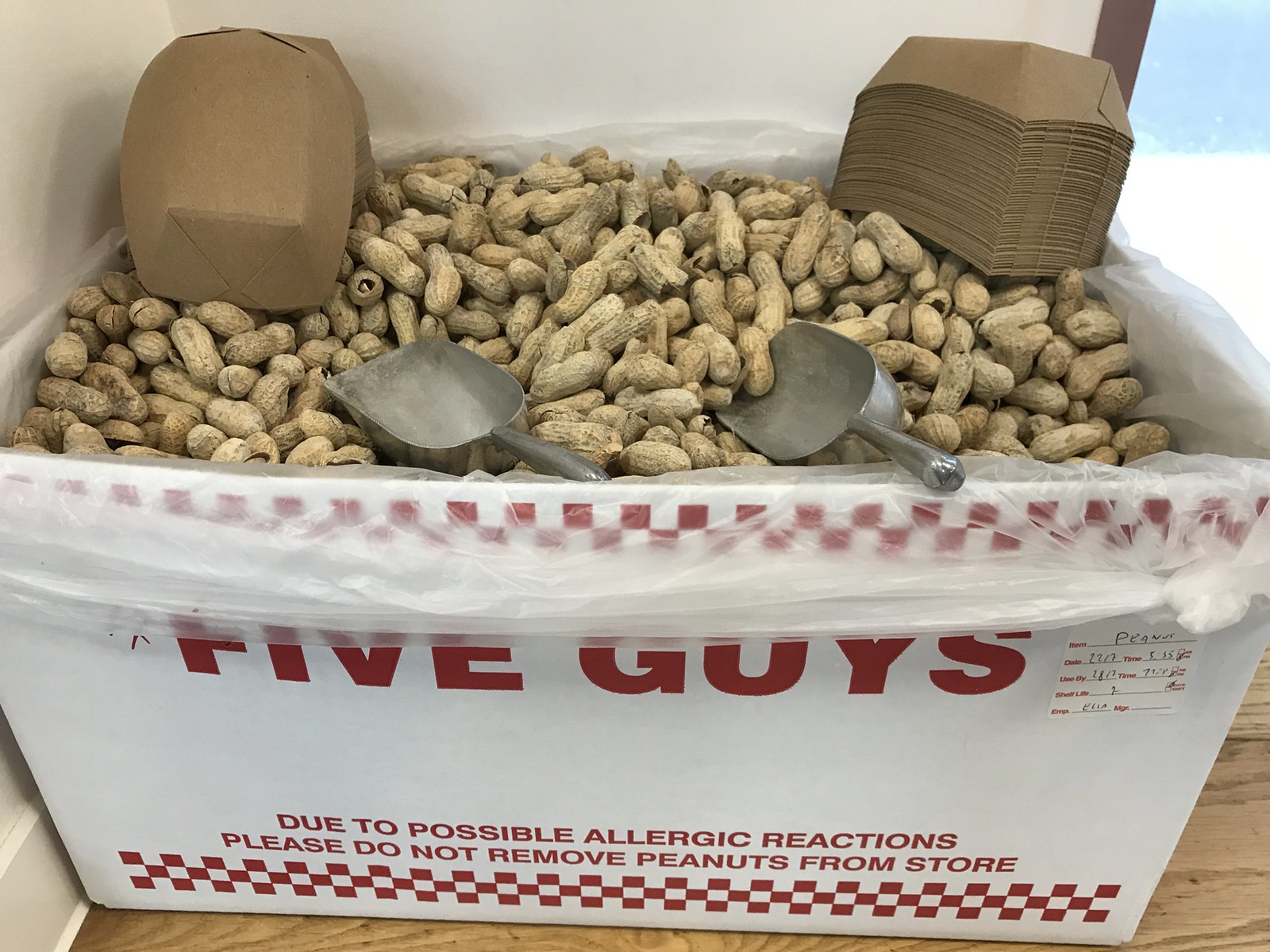The image shows a large white box labeled "Five Guys" with three rows of red and white checkerboard squares running across its top edge. Inside the box is a plastic liner, the edges of which are visible, and it is tied on the right side. The box, brimming with dried peanuts still in their shells, also contains two large metal scoops and a stack of small, brown cardboard containers meant for holding the peanuts. Prominently displayed on the box is a warning in red text: "Due to possible allergic reactions please do not remove peanuts from store." The box sits on a wooden table, and in the background, the wall is white with a partial view of a window on the right side.